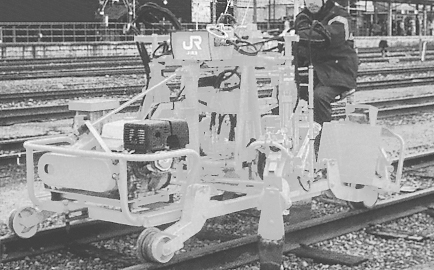The black-and-white photograph depicts a blurry but distinctive scene featuring a white metal contraption placed on railway tracks. The device, which appears to be some form of a railway maintenance tool, has four small wheels—two at the front and presumably two at the back for stability. A man, wearing a coat and seated on the contraption, seems to be operating it. The device bears the marking "J.R." and has a peculiar setup with wires and a panel on the front, as well as a gray box-like component. The scene is somewhat difficult to discern due to the brightness and blur in the image. In the background, railway tracks extend into the distance, with a fence or divider providing a stark backdrop to the mysterious machine and its lone operator.